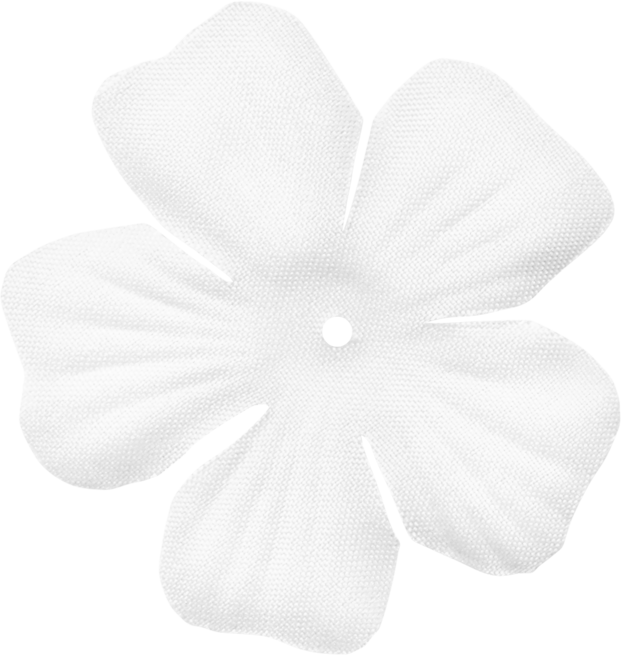This image showcases a white artificial flower, which appears to be made of cloth or fabric, set against a stark white background. The flower consists of five heart-shaped petals, each adorned with four to five subtle lines or creases that give it a more realistic texture despite its artificial nature. The petals feature a distinct fabric pattern, resembling stitching or a weave, and are slightly tilted at a 45-degree angle, contributing to its three-dimensional appearance. The center of the flower has a noticeable hole, indicative of where it would attach to a plastic stem, suggesting it might have been part of a fake bouquet or lei. Though the flower's material seems somewhat rough and on the cheaper side, its overall design manages to convey a convincing likeness to a real plumeria, especially from a distance. The petals' edges are a bit too angular and square, but they also have a natural outward curve that enhances its realistic look.